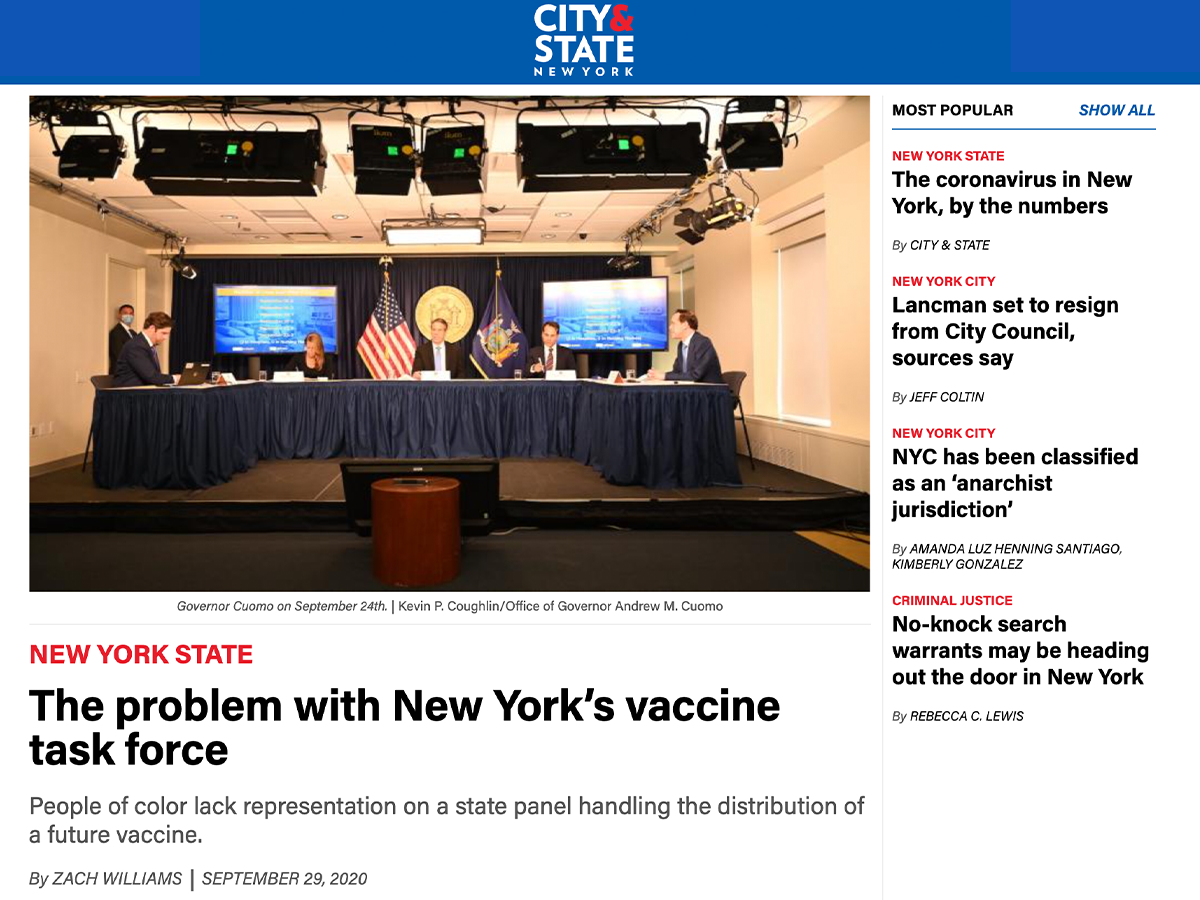The image features a predominantly white background with a distinct blue header at the top. This header showcases white text that reads "City in State, New York," punctuated by a red symbol for Anthro Sam. Below the header, there is a photograph depicting what appears to be a formal board meeting.

In the central portion of the image, a large conference room is visible, furnished with a semi-circular table draped in a black skirt. Seated at this table are several individuals engaged in discussion. Behind the person seated centrally is a gold seal, flanked by the American flag and a flag that seems to represent New York State.

The backdrop of the room includes two large flat-screen televisions. Additionally, a separate television monitor, turned in the opposite direction, is propped up against a seat. Ceiling lights with green and orange accents illuminate the room from above.

Below the image, red text declares "New York State," followed by black text that introduces an article titled "The problem with New York's vaccine task force." However, the article text is cut off. To the far right of the image, a column displays various headlines from other news articles.